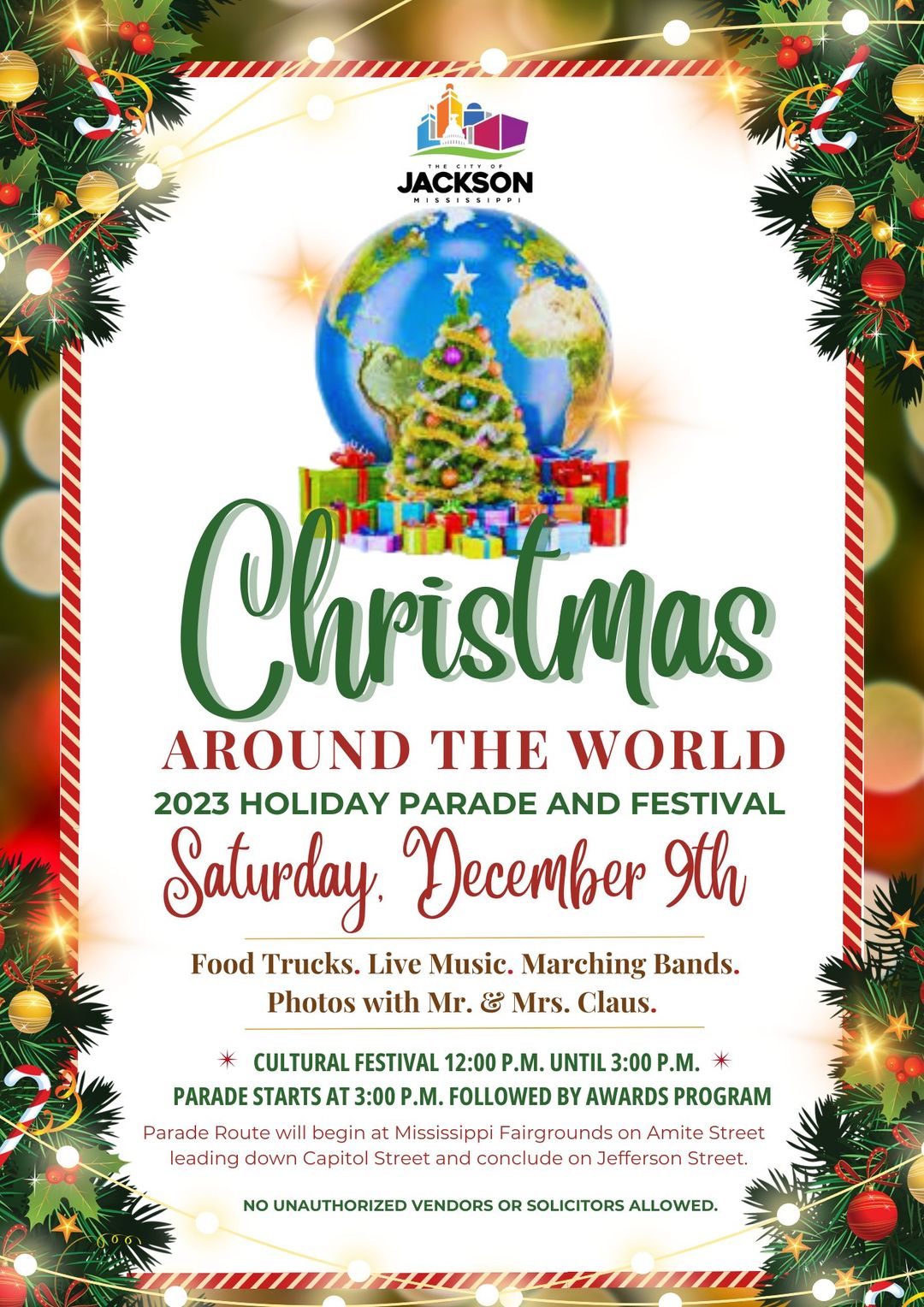The poster advertisement for the "2023 Holiday Parade and Festival" is festively designed against a backdrop of Christmas lights on either end. The border is adorned with a classic candy cane stripe pattern in red and white, framing the poster. The four quadrants feature Christmas greenery with candy canes and ornaments, including bulbs and golden-colored Christmas balls, though there’s a quirky detail in the bottom corners where the ornaments and candy canes appear reversed.

At the top, the poster is presented by a company associated with the city of Jackson, depicted with a small building and their logo. Below this, a globe symbolizes the theme "Around the World," accompanied by a decorated Christmas tree with varied colorful presents underneath. 

In bold, alternating text, the poster announces "Christmas Around the World" in green and red, followed by the event title "2023 Holiday Parade and Festival." In elegant script, it notes the date: "Saturday, December 9th." Beneath a light brown line, detailed information highlights event features including food trucks, live music, marching bands, and photo opportunities with Mr. and Mrs. Claus. The bottom of the poster provides the date, time, parade route, and a reminder in green font: "No unauthorized soliciting allowed."